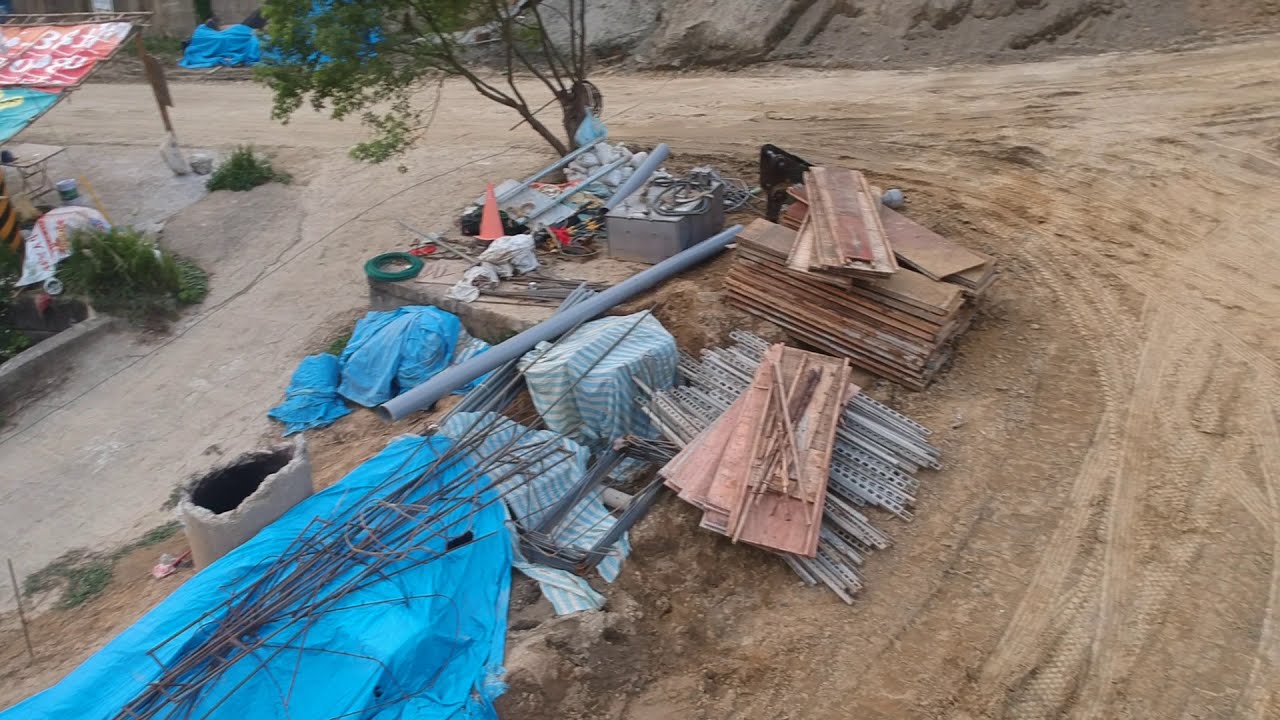The image captures a detailed, landscape-oriented color photograph of an Indian construction site viewed from a drone at approximately 10 to 15 feet in the air. The central focus of the image is a circular arrangement of construction materials scattered on a dirt terrain that bears tire tracks, suggesting recent vehicle activity. The materials, which appear messily stacked, include concrete poles, rebar, wooden planks, metal frames, large PVC pipes, and items covered with blue tarps and regular blankets. 

In the top right corner, a tent-like structure displays text in a script indicative of Indian, Pakistani, or Afghan origin. The bottom left features an orange construction cone and a bag of debris, while the left side reveals a partially visible structure with a roof made of colorful tin in red and blue, supported by a post. A small tree stands in the midst of the construction materials, adding a natural element to the otherwise industrial scene. Additional tarps and miscellaneous items are scattered throughout, contributing to the overall impression of a chaotic yet functional workspace.